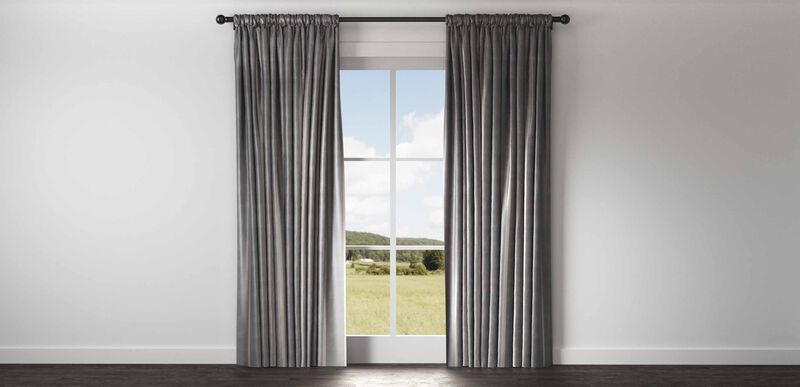The image depicts a room featuring a centrally placed, door-sized window framed in white. On either side of the window hang long, gray curtains that extend from the ceiling to the brown wooden floor. The curtains are mounted to a black metal rod fixed above the window. The walls on either side of the window are light gray, contrasting with the white light softly illuminating the floor. Through the window, a serene outdoor scene is visible, showing a vividly green grassy field, trees, and a distant mountain covered in vegetation beneath a powder blue sky dotted with white clouds. There is a subtle sense that the outdoor scene might have been digitally edited into the image, giving it an oddly perfect yet slightly artificial appearance.